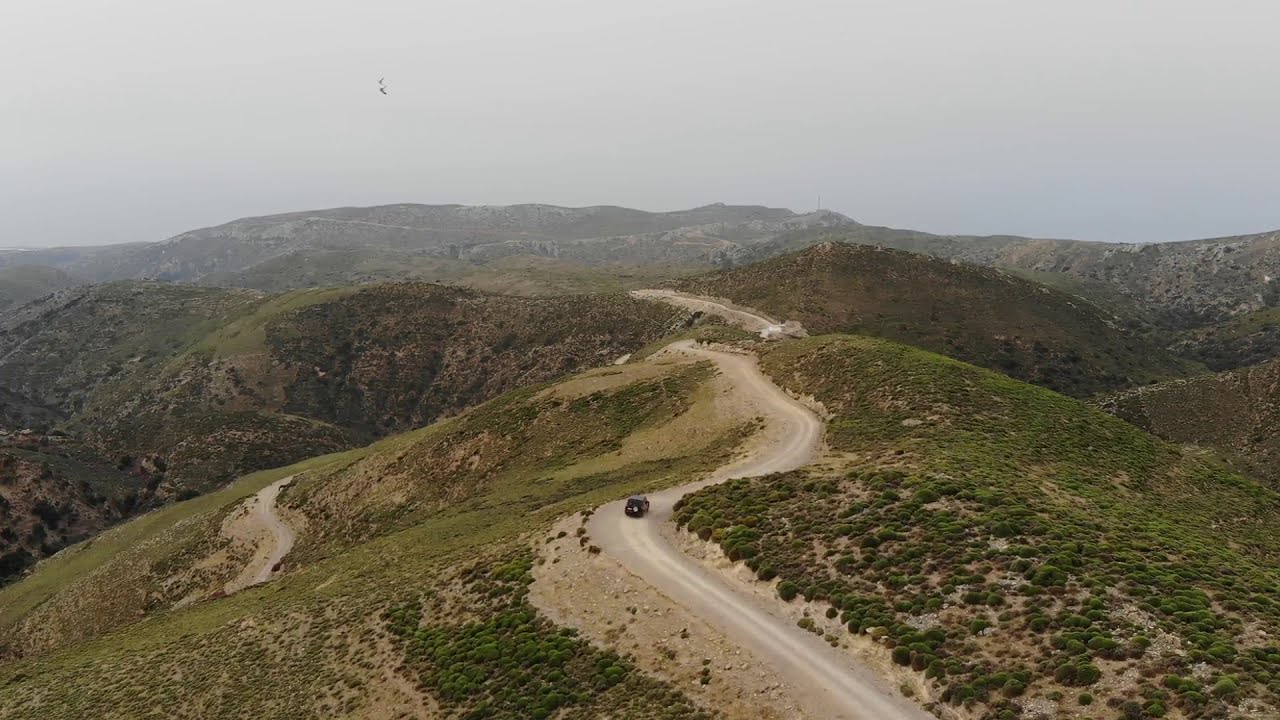The photograph captures a striking mountainous landscape with a winding dirt roadway running along the ridgeline of the hills. A solitary dark-colored vehicle, possibly a black SUV, is driving along this dirt road, which snakes its way from the bottom edge of the image to about two-thirds up where it disappears into the terrain. The hills are a mix of dark green to light green shades interspersed with patches of exposed earth, contributing to the rugged ambiance. The foreground showcases some sparse bushes and cleared dirt areas, transitioning into greener grass as the eye moves further into the scene. Additionally, there's a smaller dirt path visible at the bottom left, diverging from the main road and extending down the hill. The background reveals more rounded hills that progressively fade into a gray, hazy sky, suggesting a vast and possibly coastal expanse beyond the visible terrain.